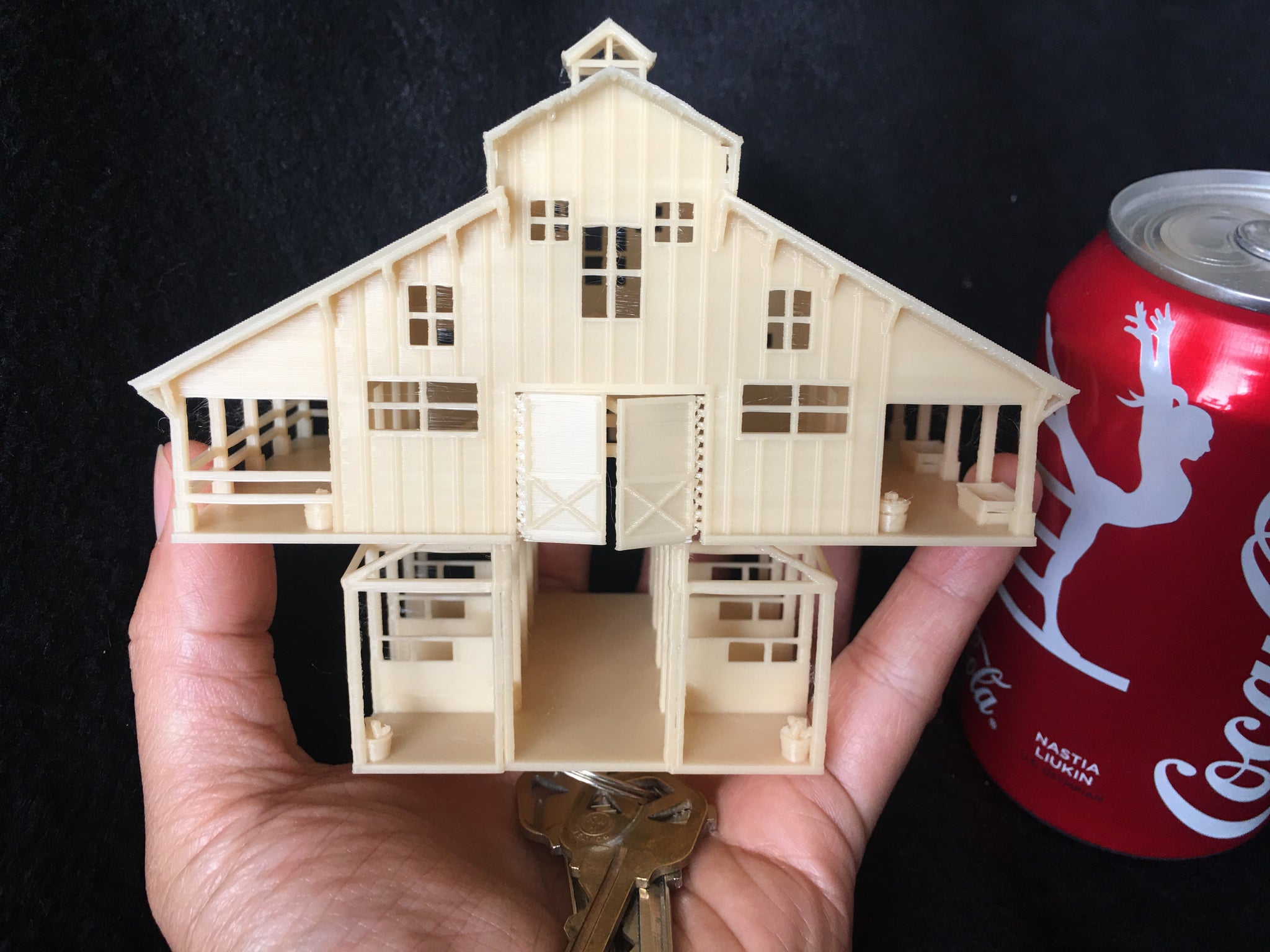The image features a detailed, miniature plastic model of a barn, predominantly white with doors at the top and a separate section resembling horse stalls at the bottom. This barn model, seemingly symmetrical with windows on both sides, is held in the left hand of a white man; in his palm lies a set of three house keys on a key ring. Adjacent to the hand, slightly off-screen, is a red Coca-Cola can with a white silhouette of a gymnast, accompanied by the name Nastia Liukin written below. The background of the photograph is a dark, blackish-blue hue, emphasizing the central subjects.